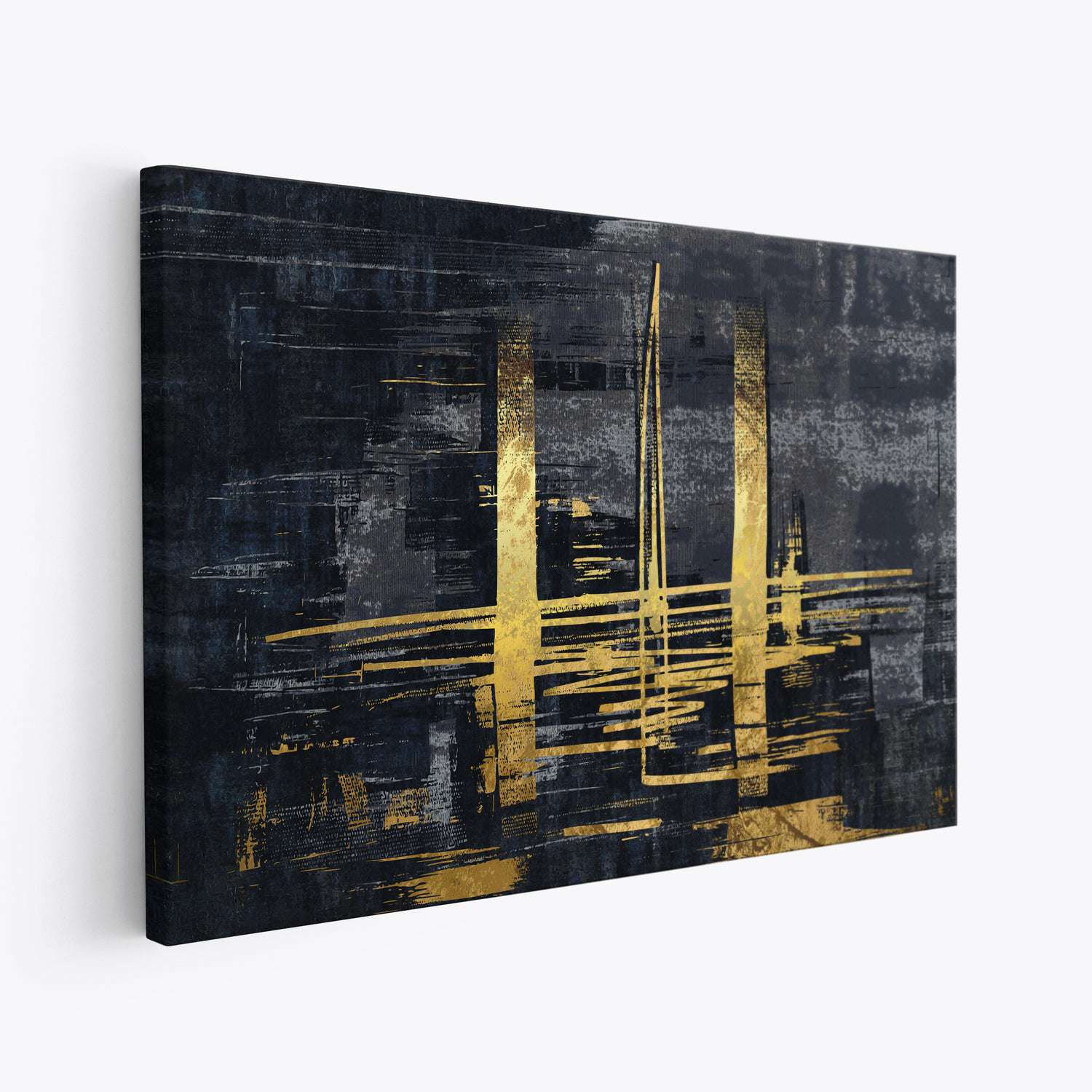The image displays an abstract painting hung meticulously on a pristine, all-white wall, evoking the ambiance of an art gallery or a meticulously maintained home. The canvas, rectangular in shape, features a grungy, gritty composition dominated by a spectrum of blacks and grays, coalescing into an atmospheric backdrop. The painting's focal point is its striking gold accents, artfully integrated to mimic the luminous quality of gold without using actual gold leaf. These gold elements include two prominent vertical lines resembling towers, a central elongated spike, and dynamic, scattered gold squiggles and strokes that traverse the canvas. The reflective gold elements suggest the impression of a bridge spanning water, with an abstract, patchworked skyline emerging behind, giving the overall image a high-fashion, urban grit. The gradient background transitions from a dark, moody black to a lighter grayish-white towards the right corner, enhancing the depth and complexity of the piece.